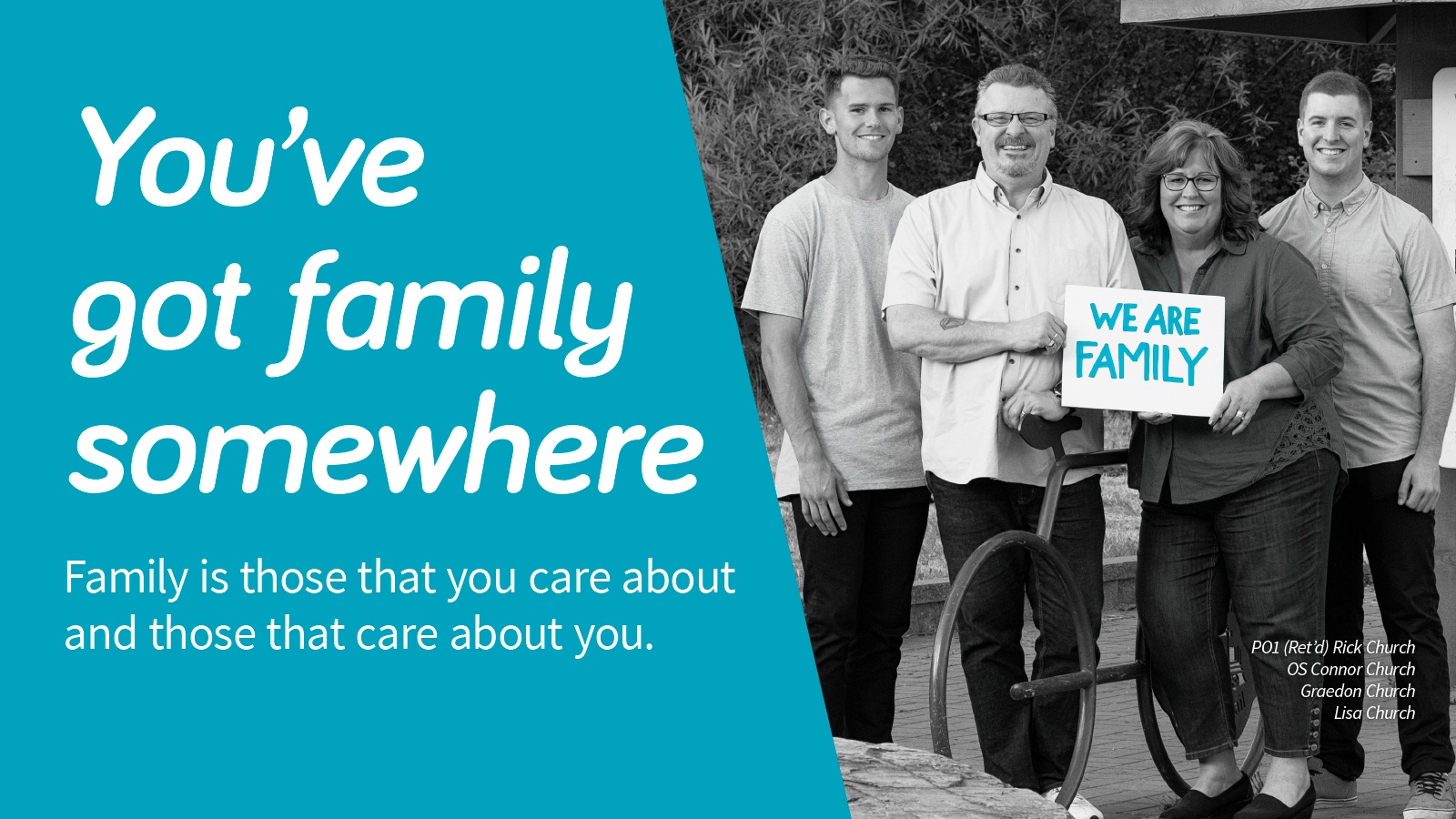The image is a horizontally-oriented rectangular visual divided into two sections. The left side features a turquoise blue background with bold, white text. The top line of text reads in large font size: "You've got family somewhere." Below this line, in smaller fonts, it states: "Family is those that care about you, and those that care about you. Family is those that you care about, and those that care about you."

The right side of the image contains a black-and-white photograph depicting a woman and three men who appear to be two younger boys and one grown man, likely a family. The woman is holding a sign that reads: "We are family." Below the photograph, additional text identifies the individuals as "PO1 Retired Rick Church, OS Connor Church, Graedon Church, and Lisa Church." The individuals, who are Caucasian, are dressed in mostly collared shirts and dark pants, with one person wearing a t-shirt. They stand around what appears to be a decorative bicycle, possibly a 10-speed, positioned as if for display, which gives the impression it could be an ornamental piece in a park.